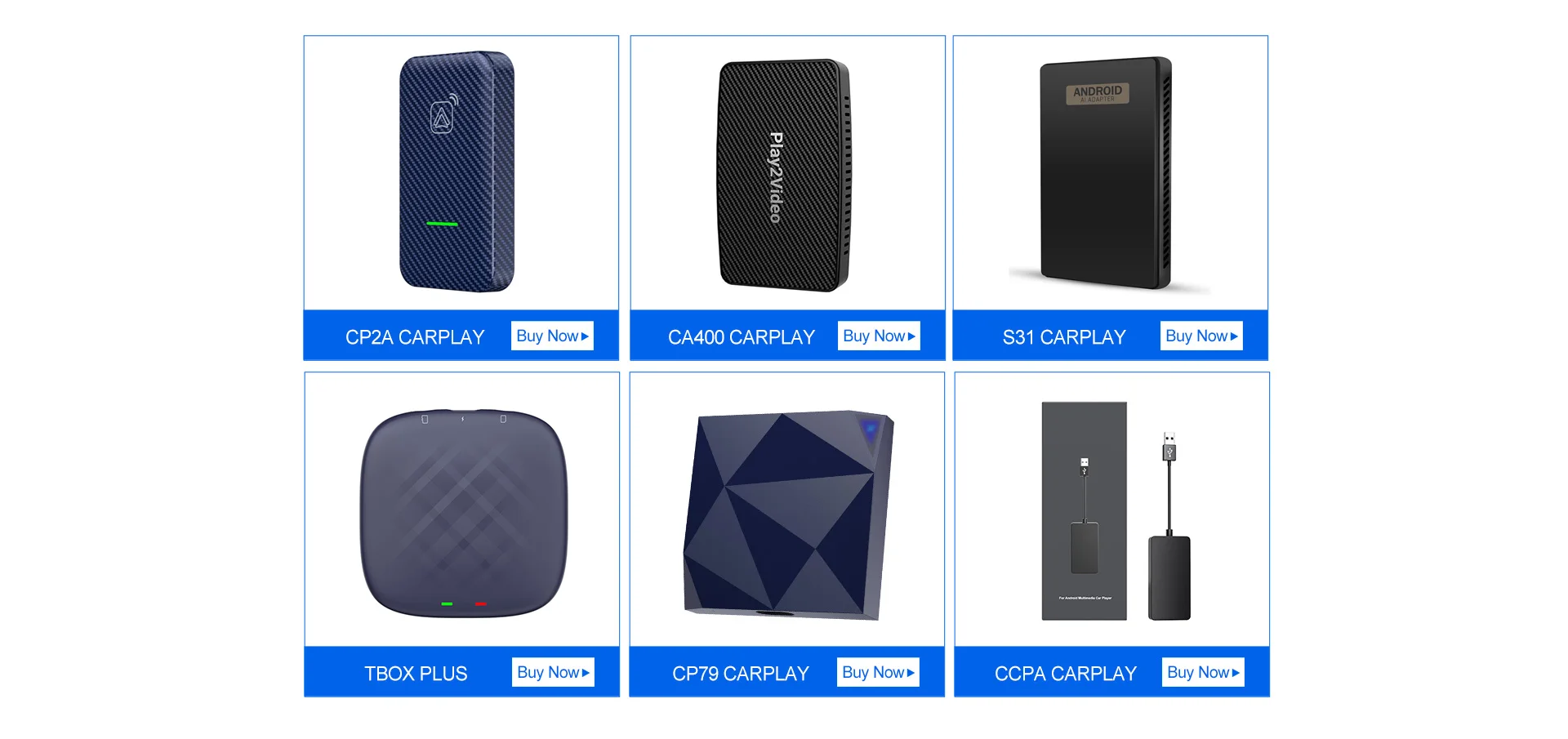The image showcases a clean, organized layout on a white background, divided into six square boxes, each displaying different types of CarPlay instruments available for purchase. Each box features a title in blue, a product image, and additional details, including buying options.

1. **CP2A CarPlay**: This section displays a sleek black box with an illuminated green light at the bottom. An inviting white "Buy It Now" button is prominently featured beneath the image.
   
2. **CA400 CarPlay**: This part showcases a box with the text "Play Video" on the front. The title CA400 CarPlay" is accompanied by a white "Buy Now" button.

3. **S31 CarPlay**: The box shown here is dark and somewhat challenging to read due to low lighting. It has a label on top, and a "Buy Now" button is present.

4. **T-Box Plus**: This square-shaped device has multiple boxes on its surface. Notably, it features both red and green buttons at the bottom, adding a touch of functionality.

5. **CP79 CarPlay**: Displaying a visually appealing, somewhat 3D black box adorned with light and dark triangles, this section also includes a "Buy Now" button.

6. **CCPA CarPlay**: This shows an image of the box with additional elements on the side, resembling a cable connection, along with the necessary buying option.

Each product is neatly presented to highlight its design and key features, making it easier for potential buyers to explore and consider their options.